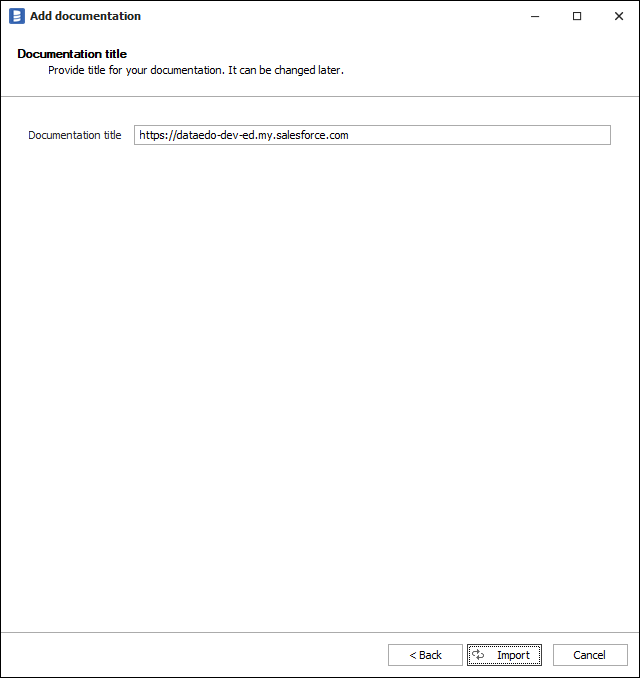The image depicts a screenshot of a computer screen focused on a web application interface for documenting within a Salesforce environment. In the top left corner, there is a blue square containing white icons and text that reads "Add Documentation." Moving to the upper right corner, standard window controls are visible, including a minimize button, a maximize/restore button represented by a square, and a close button marked by an 'X'.

Beneath the header, a section in bold text reads "Documentation Title" with a subtext, "Provide title for your documentation. It can be changed later." A faint gray dividing line follows, creating a small white space below. Underneath this space, the text "Documentation Title" appears again, accompanied by a gray text box displaying the URL "https://datido-dev-ed.my.salesforce.com".

The central part of the screen is notably blank, providing space intended for future user input or additional elements. At the bottom right corner, three buttons line up horizontally: "Back," "Import," and "Cancel," giving users navigational options within the interface.